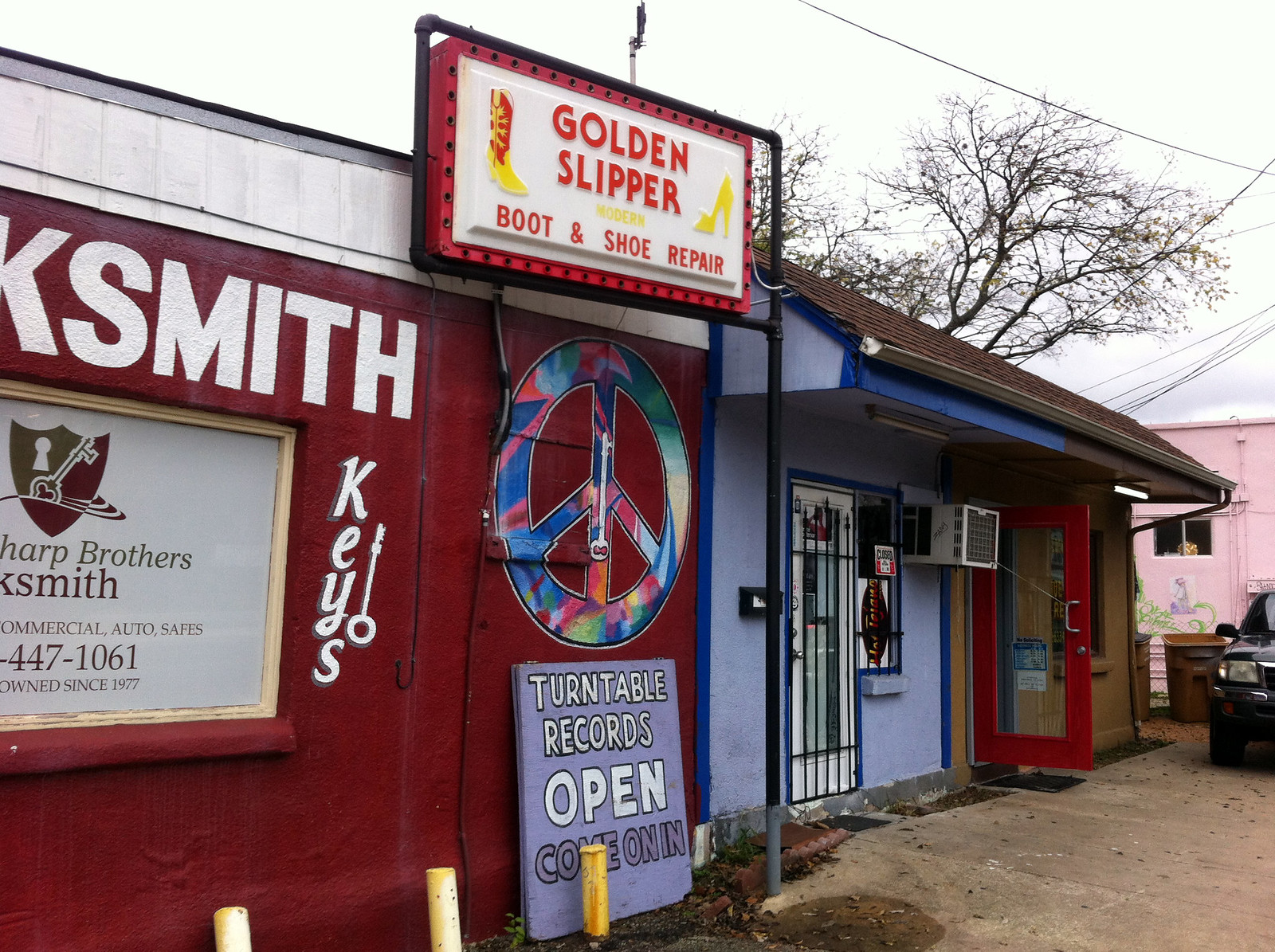The photograph captures the front of an old, rehabbed horizontal rectangular building divided into several small businesses, each with a distinct and colorful façade. On the left side, a partially visible red storefront belonging to a locksmith features white writing that reads "Keys" alongside a peace sign with a key in the center. Next to the locksmith, a larger white sign atop a blue-fronted store announces "Golden Slipper Boot and Shoe Repair," with an illustration of a cowboy boot adorning the wall. This blue store has its door open, revealing a glimpse inside. Adjacent to it is a brown building segment with an open red door, and leaning against its wall is a sign that reads "Turntable Records - Open, Come on In." The exterior area includes a concrete entranceway and a truck parked near a pink building across the yard, adding to the vibrant and eclectic atmosphere of this quaint business strip.